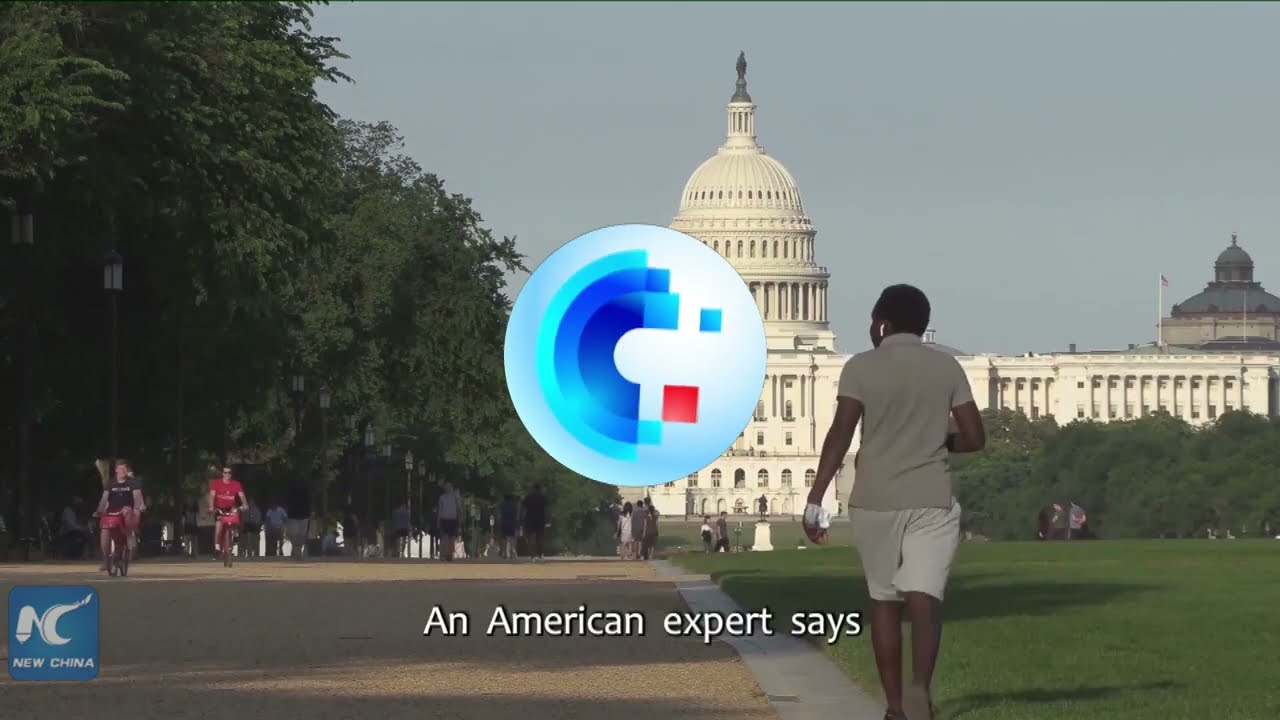This photorealistic image captures the iconic United States Capitol Building, prominently centered in the distance. In the foreground, a wide brown path lines the left side of the image, flanked by tall green trees and black, unlit light posts. This path is frequented by several people walking, running, or biking, enjoying the park-like setting on what appears to be a slightly overcast day. Among them, a Black woman in a brown khaki polo shirt and khaki shorts strides purposefully away from the camera, sporting earpods. On the right side of the image, a lush green lawn stretches towards the Capitol, dotted with more trees and individuals leisurely spending their time.

Dominating the visual space, a circular logo overlays the center of the image, featuring a stylized 'C' in light teal and dark blue, along with red and blue squares. Below this, the words "Anna Merring, Ken Expert says," are displayed in white text. Additionally, the bottom left corner of the image includes another logo—a blue square containing the white, stylized letters "NC," accompanied by the text "New China."